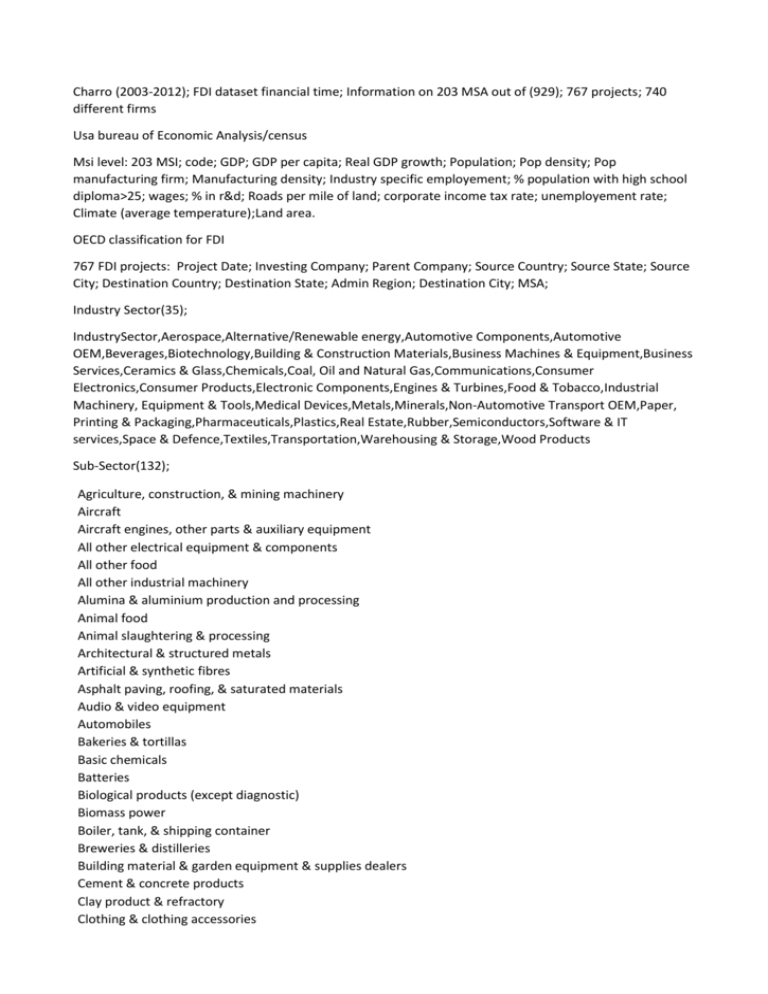"Charo: Analysis of FDI Data Set (2003-2012) - Financial Time Independence 203. This comprehensive project, MRSA 867, delves into the 740 Use of Business Ergonomic Analysis, examining various metrics such as Mix Level 203, GOP percentages, proprietary dynamics, and democratic influences in manufacturing and industrial sectors. The scientific study presents emphysema percentages, population density with high cool dioramas, and employment trends. Key findings highlight 25% wage adjustments, flood impacts per mile of land, corporate income relationships, and the correlation between late unemployment rates and socio-economic factors."